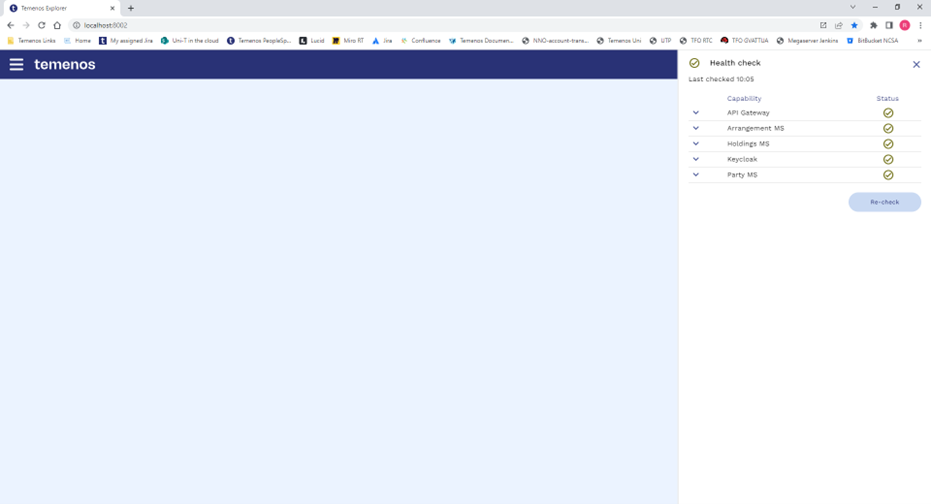Screenshot of a Google Chrome browser window displaying the "Temenos Explorer" tab at the top, with the URL set to "localhost:8002". The browser’s bookmark bar is populated with numerous saved bookmarks, including Home, Unity in the Cloud, Lucid, MiraRT, Jive, Confluence, Temenos, Uni, among others. The website's interface is largely minimalist and blank, featuring a light blue background.

On the left-hand side, a navigation bar is topped with a blue banner containing three horizontal white lines, suggesting a menu for additional options. Adjacent to this icon, the word "Temenos" is displayed. Below the banner, the page remains mostly empty.

On the right-hand side, there is a column labeled "Health Check" with an X button beside it. The page was last checked at 10:05. Listed capabilities beneath this heading include API Gateway, Arrangement MS, Holdings MS, Key Cloak, and Party MS, each marked with a green check mark icon indicating their operational status.